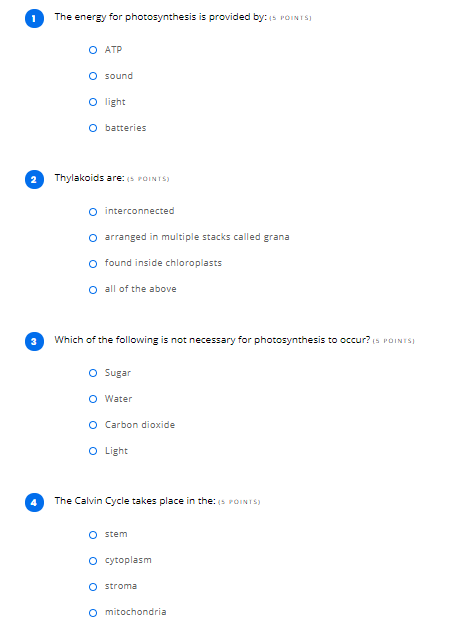This is a screenshot of a quiz focusing on photosynthesis and types of energy. The quiz page displays four multiple-choice questions, each offering four possible answers, totaling 16 points. The page has a white background with black text, and the question numbers are prominently displayed in blue circles with white numerals.

1. The first question asks: "The energy for photosynthesis is provided by?" with the answer choices being ATP, sound, light, or batteries.
2. The second question reads: "Thylakoids are?" and the options are interconnected, arranged in multiple stacks called grana, found inside chloroplasts, or all of the above.
3. The third question poses: "Which of the following is not necessary for photosynthesis to occur?" offering the choices of sugar, water, carbon dioxide, or light.
4. The fourth question asks: "The Calvin cycle takes place in the?" with answer choices being stroma, cytoplasm, stroma, or mitochondria.